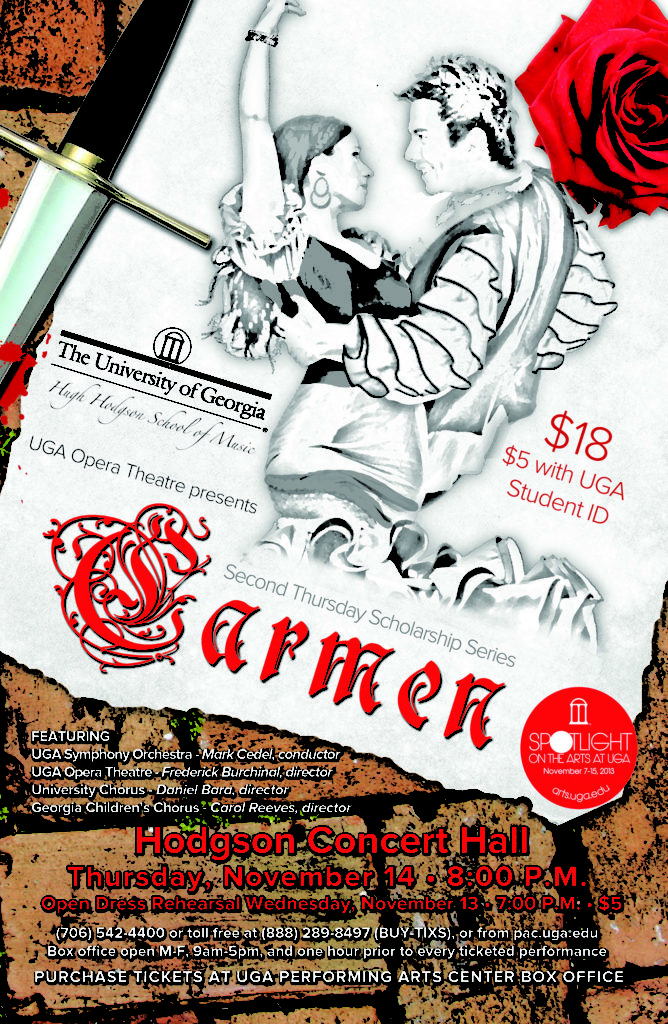This is a detailed print advertisement for a production of "Carmen" at the University of Georgia Opera House. The backdrop features a red and beige brick pattern, with a white piece of paper diagonally positioned across the top half. At the top corner of the paper, a red rose is prominently displayed. Below the rose, a vibrant illustration depicts a man and a woman in traditional flamenco-style costumes. The woman, wearing hoop earrings and a black top with a matching skirt, has her right arm elegantly raised over her head. The man, in a white striped shirt and short haircut, smiles while holding the woman around her waist.

The event details are scattered around the illustration: To the right, the ticket prices are listed as "$18, $5 with UGA student ID." Centered at the top of the white paper is an ornate "C" followed by "Carmen," and to its right, an orange circle with the word "spotlight." At the bottom, in both red and white text, the advertisement reads: "University of Georgia Hoyt School of Music UGA Opera Theater Presents Carmen, Second Thursday Scholarship Series, Featuring UGA Symphony Orchestra, Hodgson Concert Hall, Thursday, November 14th, 8 p.m." Additional details include an open dress rehearsal on Wednesday, November 13th at 7 p.m. for $5, and contact information for ticket purchases at the UGA Performing Arts Center box office. A dagger with a dark handle and a silver blade rests to the far upper left of the paper, adding a dramatic touch to the composition.